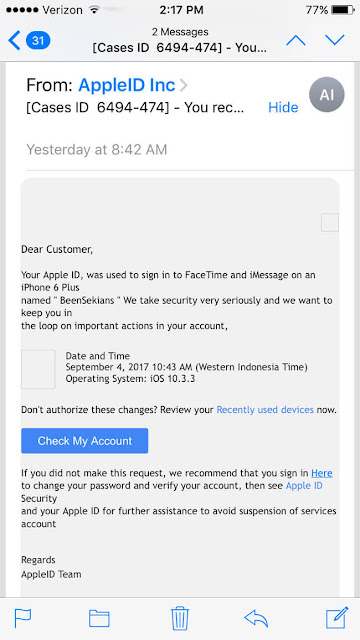**Detailed Caption:**

The screenshot captured from a mobile device displays an email sent from "Apple ID Inc," with the sender's name highlighted in blue. Below the sender's name, the email subject, enclosed in square brackets, reads "[Cases ID 6494-474] - You received..." followed by an ellipsis. Next to the subject line, the text "hide" appears in blue, and a circular bubble filled with grey and the white initials "AI" is visible. The email was sent at 8:42 AM yesterday.

The entire email is presented within a grey-sectioned rectangle with rounded corners, demarcated at the top by a thin horizontal grey line. The email content begins with "Dear Customer," and informs the recipient that their Apple ID was used to sign into FaceTime and iMessage on an iPhone 6 Plus named "Ben Sakians." The message emphasizes the importance of account security and keeping the user informed about significant account activities.

Below the introductory text, on the left, there's an empty square placeholder. To its right, the details are provided, stating:
- "Date and Time": September 4th, 2017, 10:43 AM (Western Indonesia Time)
- "Operating System": iOS 10.3.3

A prompt warning follows: "Don't authorize these changes? Review your recently used devices now," where "recently used devices now" is highlighted in blue.

Underneath this warning, the email contains a blue rectangular button with white text labeled "Check My Account." The final advisory message encourages the recipient to change their password and verify their account if the request wasn't made by them, mentioning "Apple ID security and your Apple ID" for further help to avoid service suspension. The email concludes with "Regards, Apple ID team."

At the bottom of the screenshot, five email action icons are displayed against a grey background: a blue flag, a blue folder, a blue trash can centered between the other icons, a blue forward arrow, and a blue compose new message icon.